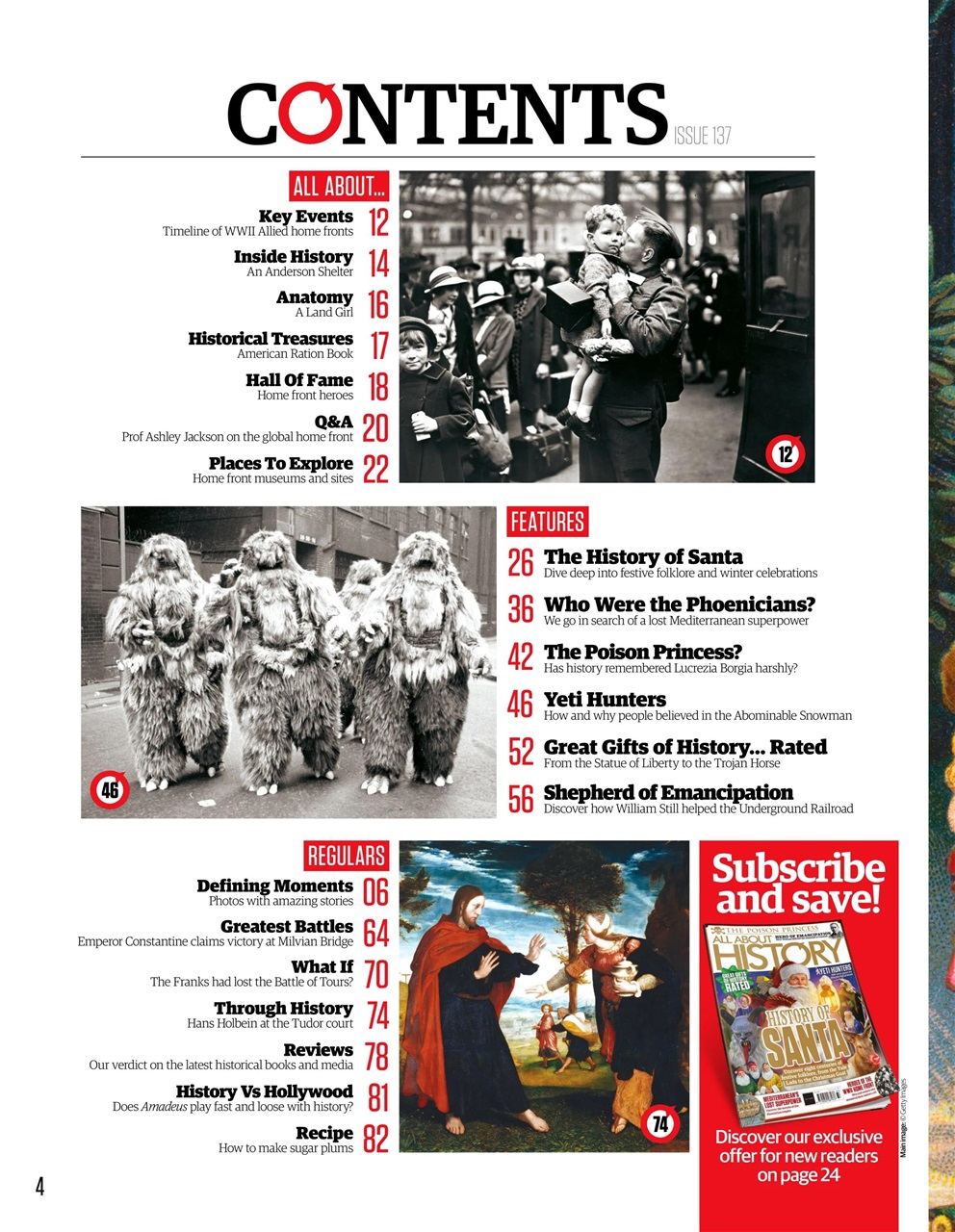This is a detailed description of an image of the Table of Contents page from a book. At the top, the word "Contents" is prominently displayed in bold print. Interestingly, although the word is in black, the letter "O" stands out in red and features an arrow circling around it, drawing special attention to that section.

Adjacent to the title, the page denotes "Issue 137," indicating the specific edition of the book. Further down, the layout is organized with textual content aligned on the left side while the corresponding visual images are placed to the right. As you scan down the page, this pattern continues, with text describing the contents and images enhancing the layout.

At the very top of the page is a rectangular box filled with red, with white print inside that reads "All About..." followed by ellipses. Below this, the contents are arranged by page numbers, which are colored in red, with descriptive titles printed in black. For example:

- On page 12, there's a section titled "Key Events Timeline of World War II."
- On page 14, the "Allied Home Fronts" content is listed.
- Page 16 features an article under "Inside History" about the Anderson Shelter.
- "Anatomy of a Land Girl" is on page 17.
- "Historical Treasures" can be found on page 18.
- The "Hall of Fame" section is on page 20.
- A Q&A segment is listed on page 22.
- Places to Explore are detailed further down the line.

This layout likely continues similarly throughout the page, blending informative text with relevant imagery.